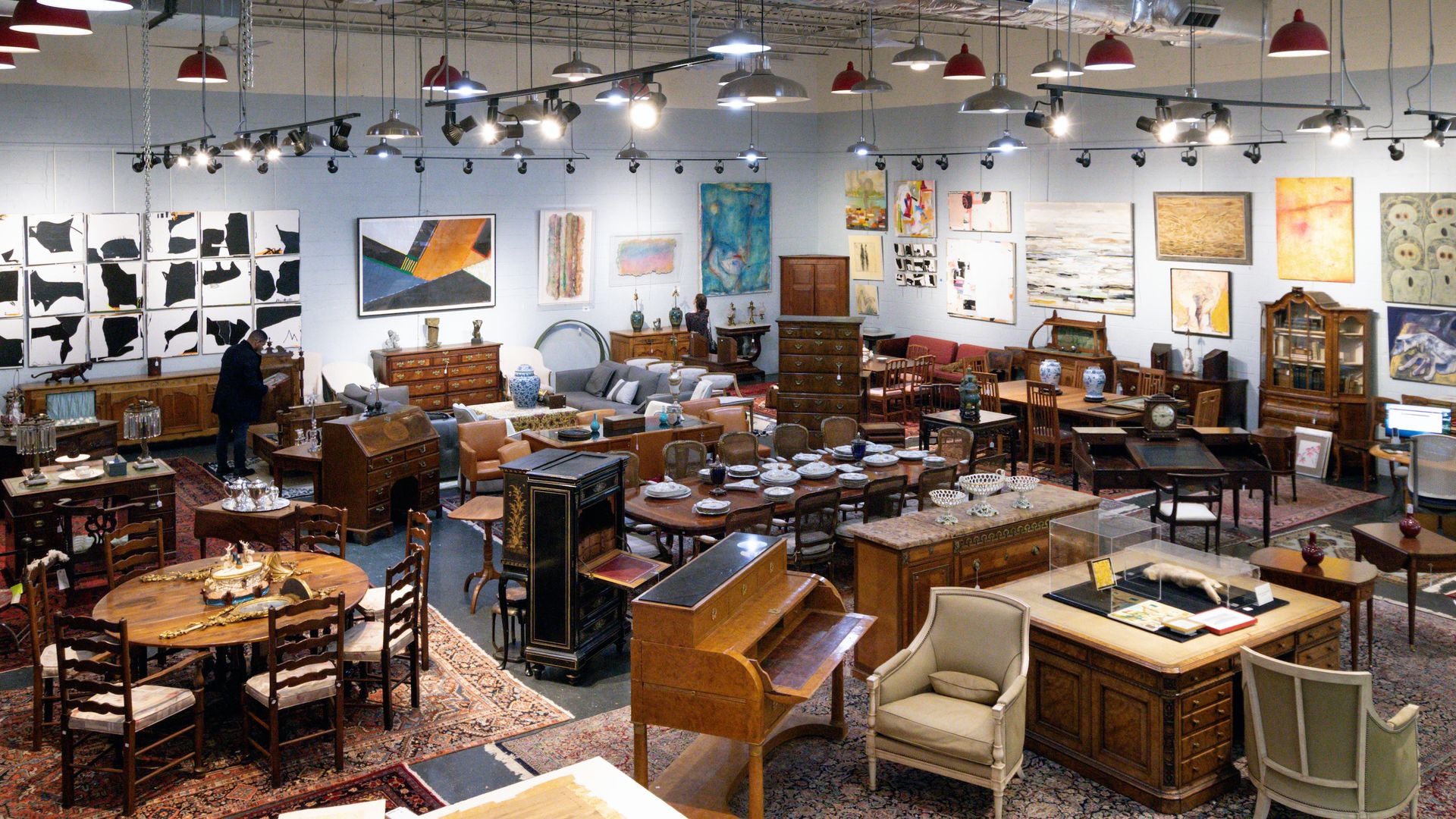This color photograph captures a spacious furniture showroom, likely second-hand, filled with an eclectic mix of vintage and modern pieces. The background features light gray, or possibly pale blue walls, adorned with various modern art paintings. Overhead, a multitude of brightly lit, dangling lights in red, blue, and green hues, appear like upside-down megaphones, illuminate the scene. The furniture, arranged both up against the walls and in the center of the room, includes an array of tables with table settings, chairs, desks, side desks, chests of drawers, coffee tables, armchairs, and possibly a piano. The rectangular composition of the photograph, taken from a slight upward angle, adds to the sense of depth and crowdedness, highlighting the diverse assortment of items on display. The casual, somewhat dated nature of the photo suggests it was taken by an amateur photographer.